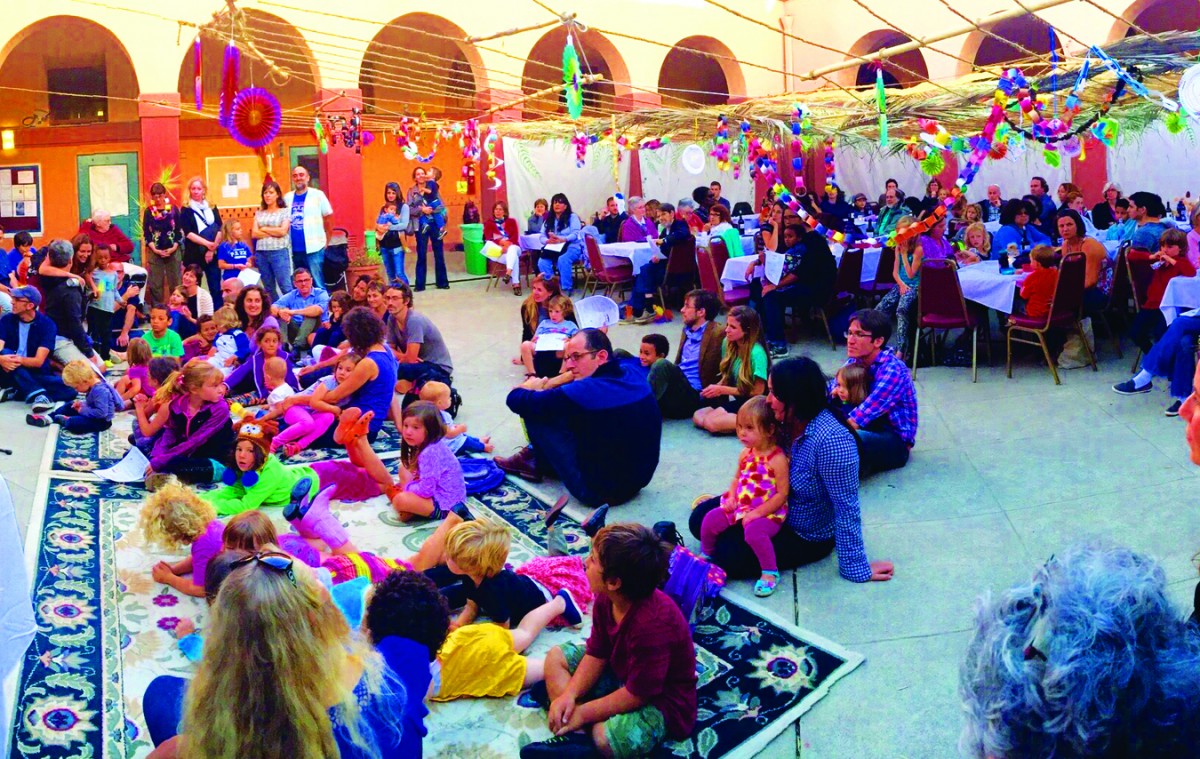This photograph captures a large, open indoor space buzzing with communal activity. The scene is centered around a group of approximately 20 children and a few adults seated or lying down on blue-bordered, white-center rugs that dominate the foreground. These rugs extend towards the left, defining a cozy, intimate ground-level space for the youngest attendees. Surrounding this area, particularly to the right and in the background, numerous tables covered with white tablecloths and red chairs are strategically arranged, accommodating an assorted group of adults who are either seated or standing.

The backdrop features walls painted in an orange-peach hue, punctuated by five visible archways, with three additional arches observable along the right wall. Adding to the festive atmosphere are the decorations strung across the room. Colorful paper chains hang in a U-shape from strings suspended above, reaching from the right side over the tables towards the left, nearly to the center of the image. Further adorning the ceiling space are round paper fans contributing to the vibrant scene. Behind the tables, white drapes add a soft, elegant touch to the background, completing the celebratory ambiance of the gathering.